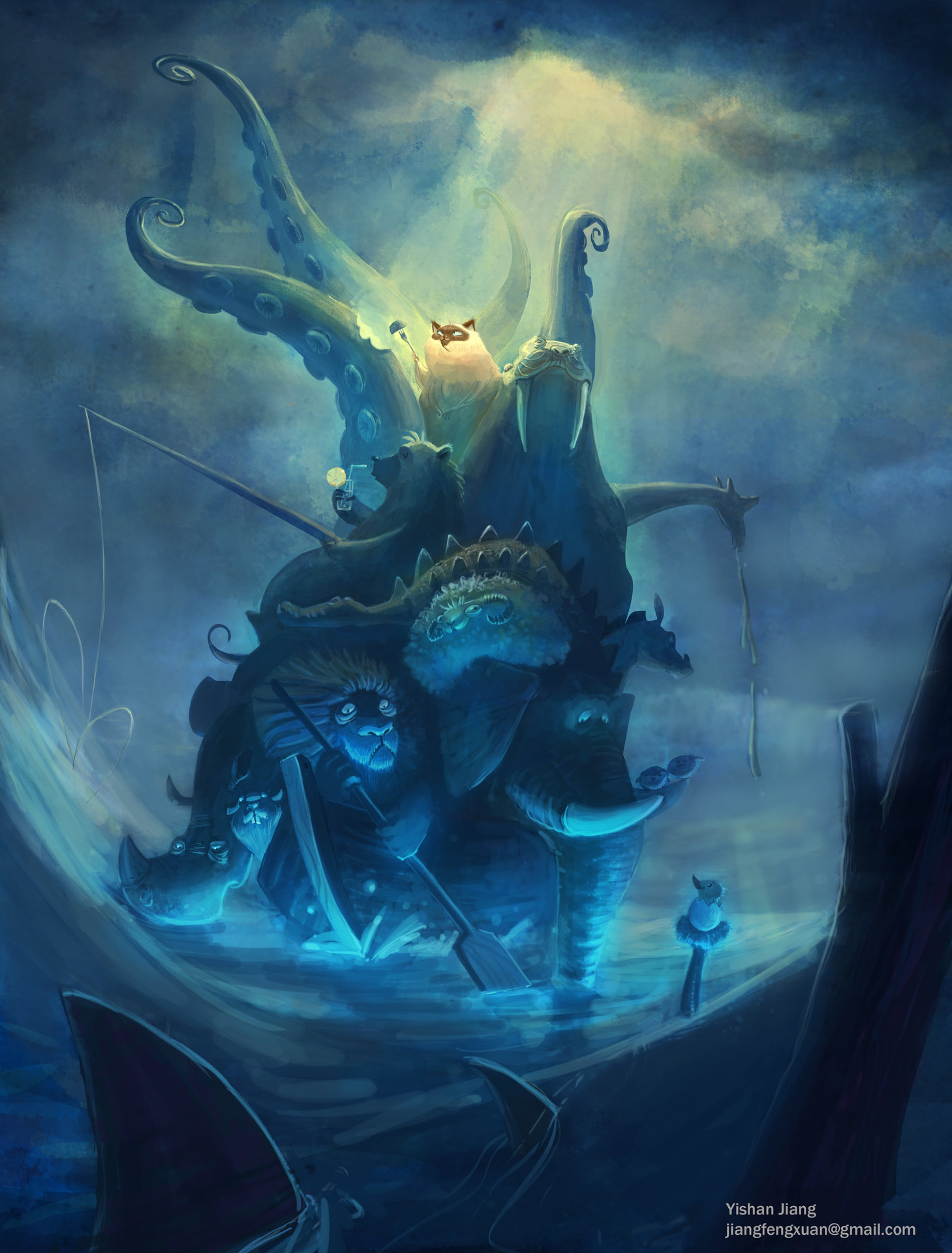The fantasy illustration showcases a surreal scene, painted primarily in varying shades of blue with touches of green and white. Central to the image is a towering boat-like structure composed of an amalgam of fantastical creatures. At the helm, a lion wields an oar as if rowing the peculiar vessel through the water. Mirroring this fantastical voyage, a massive grizzly bear lounges against a walrus, both part of the ship's hull. Above them, a white Siamese cat sits majestically, its silhouette highlighted by a shaft of sunlight piercing the cloudy sky. 

Complexity abounds as a chaotic assemblage of animals extends from the vessel: an elephant's trunk reaches down into the water, while a mischievous giraffe stretches its neck out to the right, overlapping with the dark blue tentacles of an octopus. The scene grows eerier with the presence of a rhinoceros peering over the edge and shark fins slicing through the churning waves below. Birds rest on the elephant's tusks, adding a touch of calm to the turmoil.

The entire tableau is framed on the right by a branch, and at the bottom right corner, the artist’s name and email, "Yishan Jing," are inscribed in tiny white font. The filled composition invokes the notion of a fantastical Noah’s Ark, traversing a mythical ocean under the celestial spotlight.